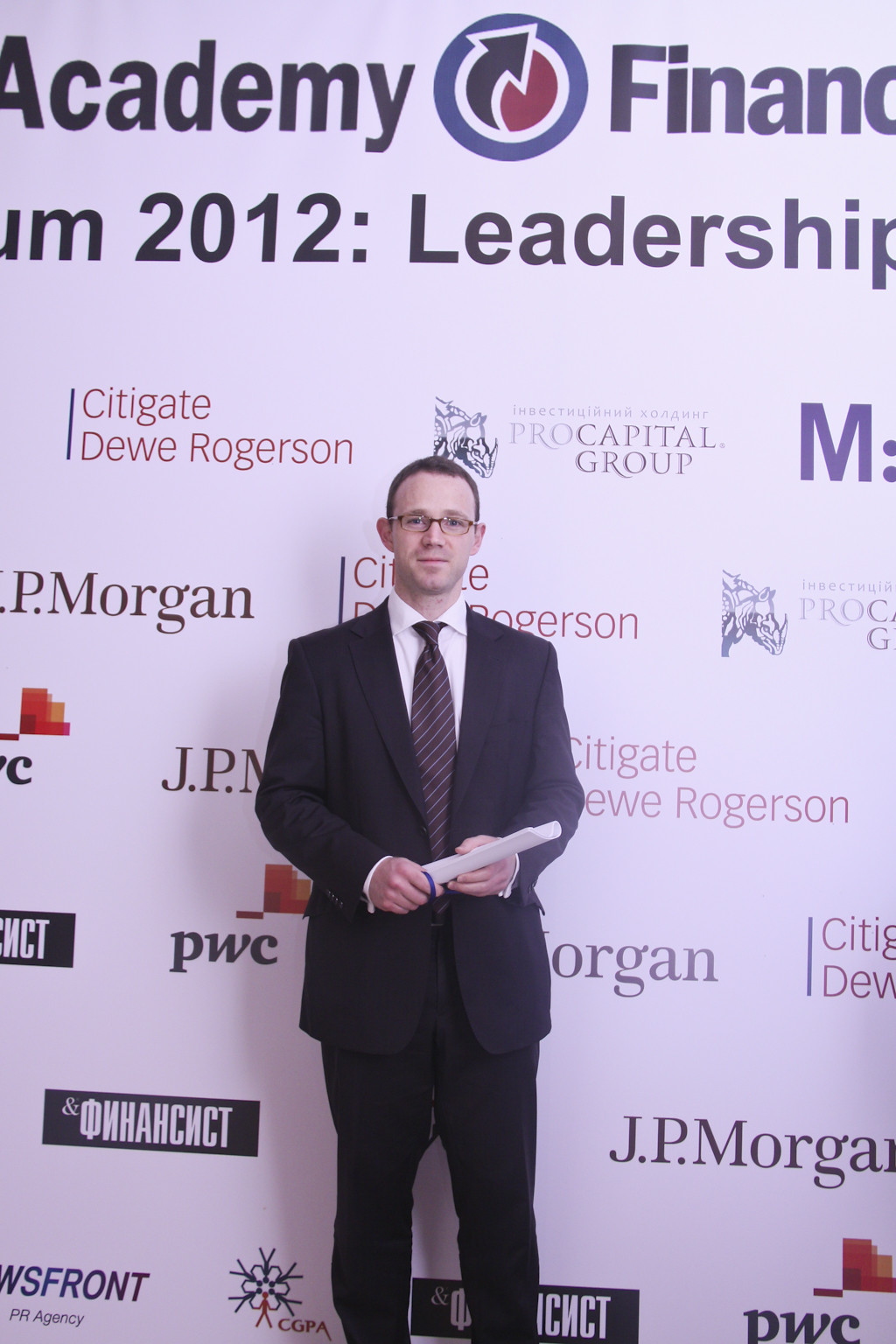The image features a Caucasian man standing against a white backdrop adorned with various words and logos, suggesting a formal event or gathering, possibly a conference or celebration. The backdrop prominently displays partial text including "Academy," "Finan..." with the remainder cut off, and "2012 Leadership." Additionally, logos and names of financial institutions like J.P. Morgan, Citygate, Dew, Rogerson, Pro Capital Group, and one written in Russian are repeatedly visible. The man, positioned centrally, is attired in a dark suit, striped tie, and white dress shirt. He has short brown hair, wears glasses, and holds some folded white papers in his hands.